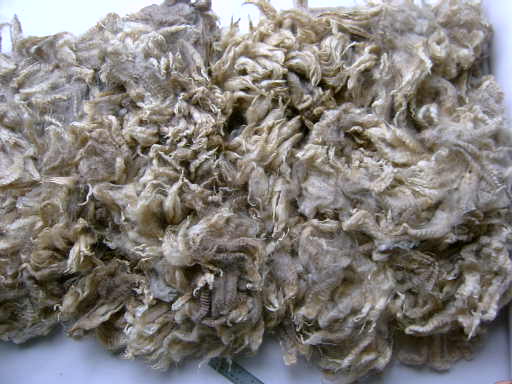The image depicts a close-up view of freshly sheared wool haphazardly piled together, displaying a mix of white, tan, and brown colors with hints of gray. The wool appears matted and intertwined, similar to the innards of a used, discolored cigarette filter or clippings from a hairy animal like a lamb or dog. The photograph captures the golden brown, dirty blonde hues of the wool on a white table, against a white wall, with a ruler placed near the center bottom for scale.